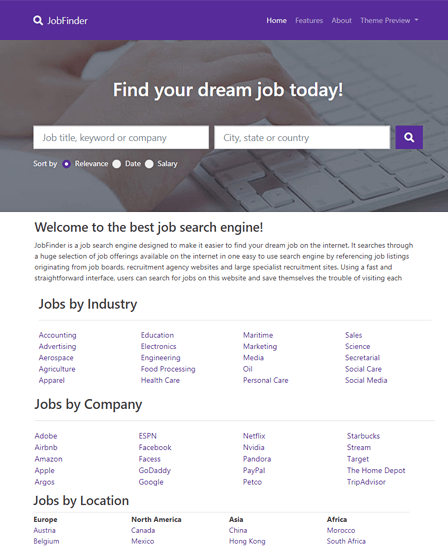This is a screenshot of a Job Finder web page. At the top of the page, a horizontal blue or purple banner stretches across the screen. In the top left corner of the banner is a magnifying glass icon, followed by the text "Job Finder." 

On the far right side of the banner, the navigation options read "Home," "Features," "About," with "Theme Preview" offering a drop-down menu. Below the banner, a photograph depicts a person typing on a white keyboard. Their hands, which are light-skinned and wearing white sleeves, enter the frame from the lower left-hand side, while the keyboard occupies the right side of the image. 

Beneath the photograph, bold text reads, "Welcome to the Best Job Search Engine." A paragraph below this headline explains that Job Finder is an advanced job search engine designed to streamline the process of finding one’s dream job online. It aggregates job listings from various sources, including job boards, recruitment agencies, and specialist recruitment sites, offering users a straightforward, fast interface that saves time and effort.

At the bottom of the screenshot, there are organized sections titled "Jobs by Industry," "Jobs by Company," and "Jobs by Location," providing users with easy access to a wide array of job opportunities.